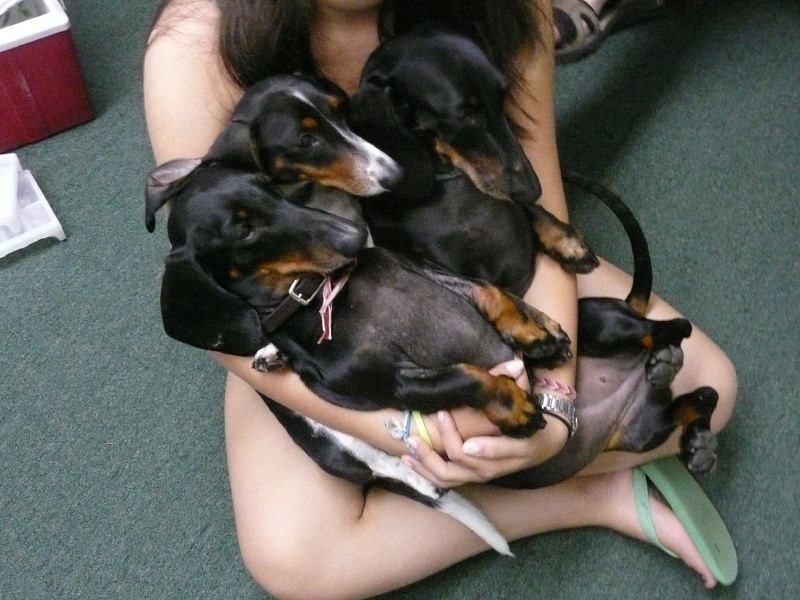In this slightly blurry, landscape-mode photograph, a woman sits cross-legged on a dark turquoise carpet, holding three small dogs that appear to be dachshund mixes. The woman, wearing green flip-flops, has her arms wrapped around the black dogs, each of which features brown and white markings. Their bellies face upwards, and their heads are turned towards the right side of the image. The woman’s hair cascades over her shoulders, and she wears bracelets and a watch on her wrist. The dogs are adorned with brown leather collars with silver buckles, and their front paws rest on the woman's arms as they lie smushed together in a row. In the background, a cooler can be seen at the top left corner of the image. The intimate arrangement highlights the close bond between the woman and her adorable, floppy-eared companions.